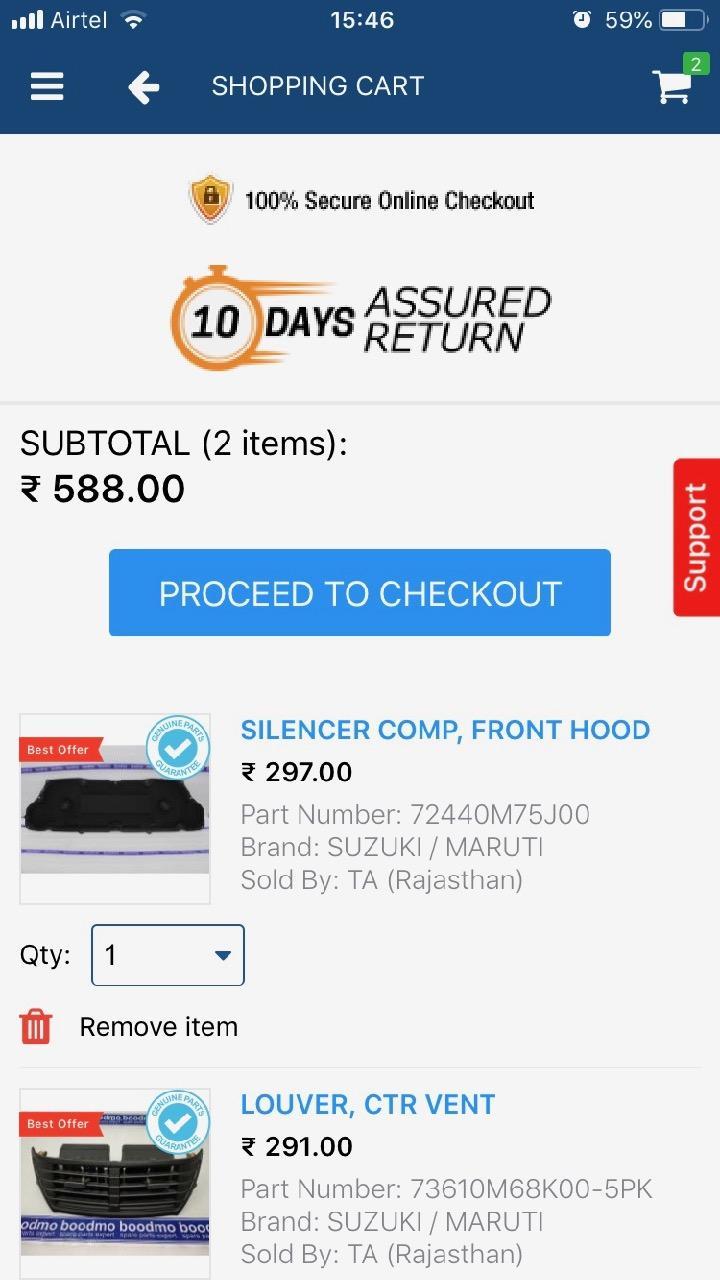A screenshot of an online shopping site is displayed on a mobile device. At the top of the screen, the status bar is visible, showing the signal strength with four bars, the carrier "Airtel," the time "15:46," and a battery indicator at 59% charge. Below the status bar, there is a navigation arrow labeled "Shopping Cart" on the left, and a shopping cart icon on the far right with the number "2" above it, indicating two items in the cart.

Underneath, there is an icon of a shield with a lock, accompanied by the text "100% secure online checkout." Next, an icon of a stopwatch with a "10" inside it is followed by the message "10 days assured return." Further down, the text "Subtotal, 2 items, 588.00" is displayed, followed by a blue rectangular "Proceed to Checkout" button.

On the far right side of the screen, a vertical red box labeled "Support" runs up and down.

The first item in the cart is detailed below, reading "Silencer Comp, Front Hood, 297.00," with a part number "72440M75J00," branded "Suzuki/Maruti," and sold by "TA, Rajasthan." The item quantity is "1," selectable via a dropdown menu, next to a trash can icon labeled "Remove Item."

The second product listed is a "Luver CTR Vent" priced at "291.00," also featuring its part number, brand, and seller information. Both items have images associated with them.